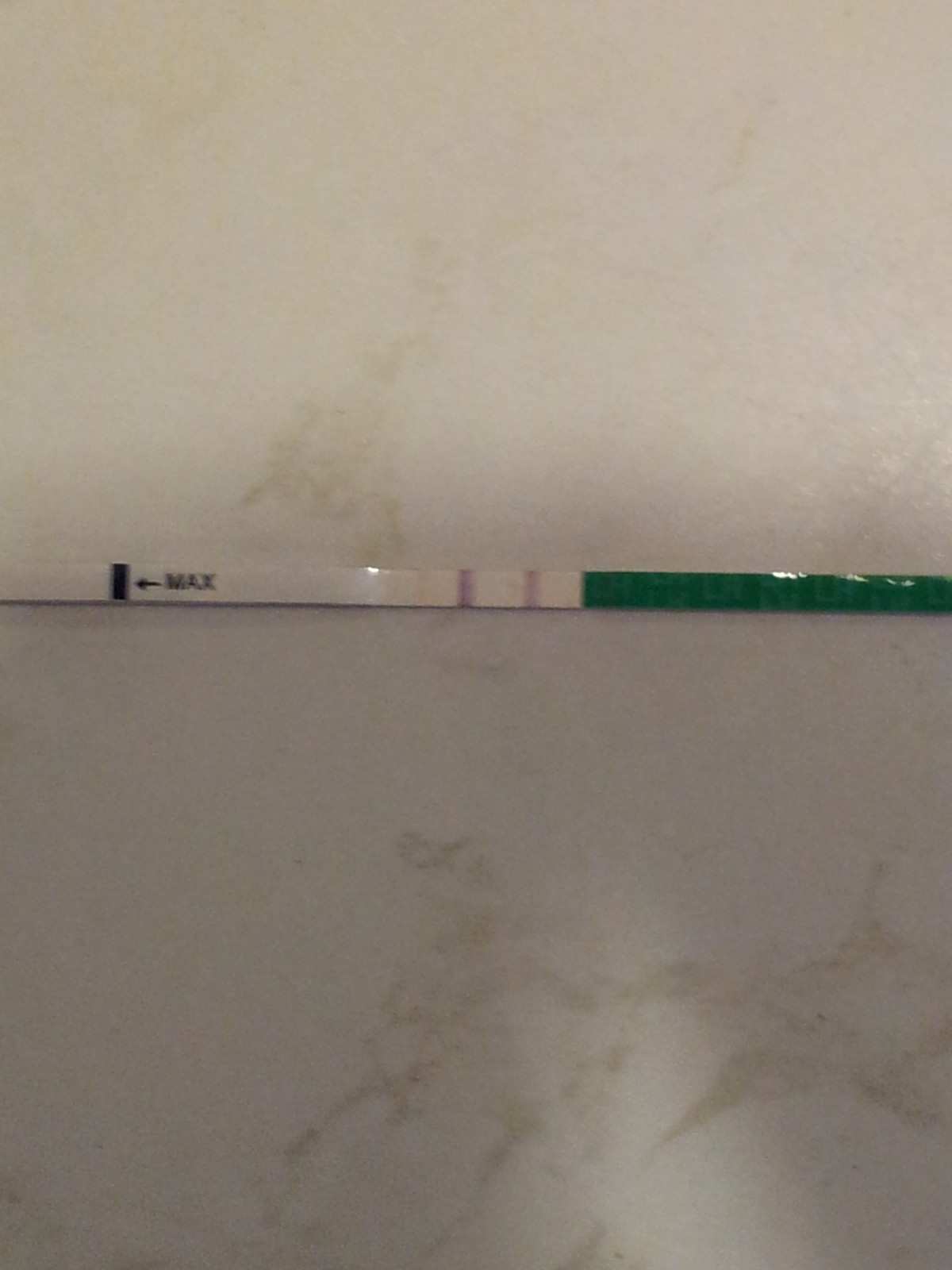The image showcases an interior wall with a horizontal strip of tape applied across it, extending from left to right. The wall itself features an off-white surface with intricate, marble-like designs and patterns rendered in a light greenish-gray color, giving the wall a textured and elegant appearance. The tape, which has a glossy and shiny finish, appears slightly out of focus, obscuring some of its more intricate details. The left portion of the tape is white, transitioning to green from the midpoint to the right edge. On the white section of the tape, a black arrow points leftward towards a black strip, accompanied by the word "marks." The green portion of the tape contains various measurement markings and numerical indicators. Overall, the tape adds an element of contrast and functionality against the patterned wall surface.